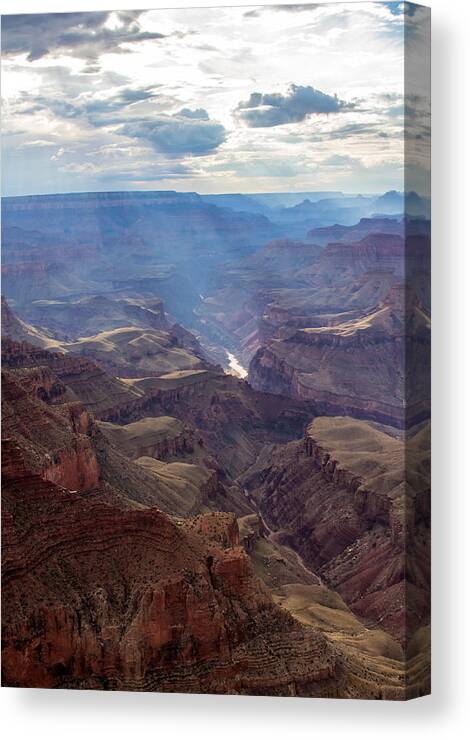The image depicts a detailed painting of a mountainous landscape, wrapped around a three-dimensional canvas frame. The scene is reminiscent of the Grand Canyon, showcasing steep, reddish-brown rock formations with distinct layers of horizontal strata. A sinuous valley cuts through the middle, originating from the bottom right and meandering upward, partially obstructed by rocky outcrops. In the background, blue and gray mountains rise towards a horizon capped by a pale, white sky filled with dense clouds, some with darker undersides. Sunlight streams through the cloud cover, illuminating sections of the rugged terrain. Atop some of the rocky formations, patches of light olive-green grass or foliage add a touch of verdant color. The painting is so detailed that it even extends onto the painted sides of the canvas, providing a fully immersive visual experience.